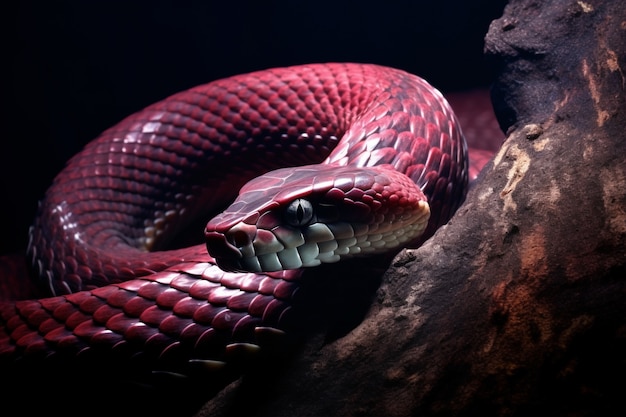In this striking and highly detailed close-up image, we observe a cobra set against a pitch-black background, suggesting it is nighttime. The snake's body is intricately coiled, creating a circular form with its head extending to the left. Its scales glisten with a dramatic mix of red and black splotches, while parts of its head feature a contrasting silver coloration. The menacing eyes are described variously as black with a slanted pupil, and a grey hue with a black slit, adding to its intimidating appearance.

The lighting in the picture casts an intense spotlight on the subjects, highlighting the textures and colors exquisitely. Beneath its mouth, the cobra's chin showcases a subtle tan or white hue.

To the right of the coiled snake, a piece of wood or perhaps a rock formation is visible. This object is characterized by dark grays, blacks, and white patches, along with hints of pink and beige, which stand out under the focused lighting. The logs appear to have streaks of dark brown with white areas, contributing to the natural, yet dramatic setting in which the cobra appears to be poised to strike.

Overall, the image combines elements of surreal design with naturalistic detail, capturing the cobra in an intense, stylized fashion that draws attention to its formidable beauty and the eerie, dark environment it inhabits.